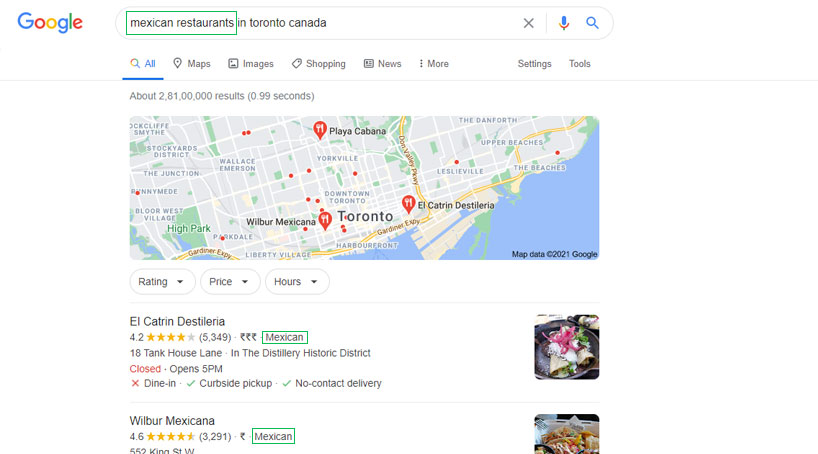A screenshot of Google Maps search results is displayed on a white background, with the distinctive Google logo positioned in the top left corner. Despite the slightly low resolution causing the text to appear blurry and grainy upon zooming in, the key details remain discernible.

At the top of the image is the Google search bar, where the user has entered "Mexican restaurants in Toronto, Canada." This query is encased in a green rectangle, emphasizing the search term. Below the search bar, the various menu options are visible: "All," "Maps," "Images," "Shopping," "News," and "More." The "All" option is highlighted in blue, indicating it is currently selected. On the right-hand side, the "Settings" and "Tools" options are also present. 

The search has yielded approximately 28,100,000 results in about 0.99 seconds. Moving further down, a map of Toronto is shown, outlining the city's edges and including blue water bodies. Several notable locations are highlighted on the map, including Playa Cabana and El Catrin Destileria, alongside numerous red dots marking additional points of interest.

Beneath the map, the top search results are listed. The first result features El Catrin Destileria, noted for its 4.2-star rating from 5,349 reviews. The listing details the restaurant as Mexican cuisine, located at 18 Tankhouse Lane in the Distillery Historic District. The status indicates that it is currently closed, with an opening time of 5 p.m. The services highlighted include dine-in, curbside pickup, and no-contact delivery options.